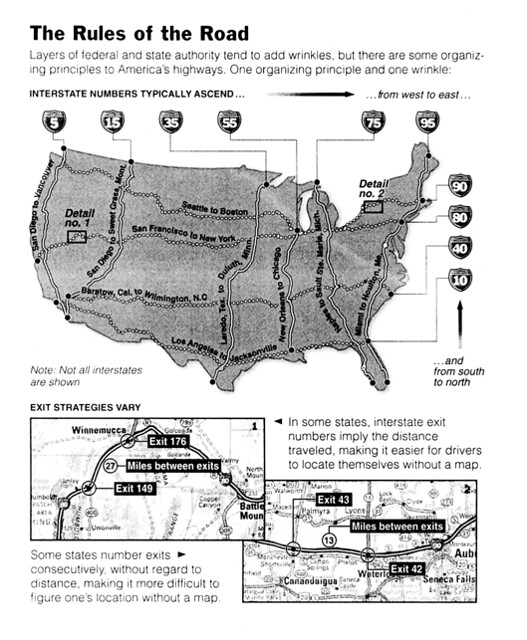This black-and-white illustration features a map of the United States with a heading that reads "The Rules of the Road." The text beneath the heading explains how layers of federal and state authority can complicate road governance but mentions that some organizing principles help simplify America's highways. One notable principle is that interstate numbers generally ascend from west to east and south to north. The map prominently displays key interstates, including I-5, I-15, I-35, I-55, I-75, I-95, I-10, I-40, I-80, and I-90, with white lines marking their routes. Not all interstates are shown. The illustration highlights that in some states, exit numbers correspond to the distance traveled, aiding drivers in navigation, while in others, exit numbers do not follow this pattern, making it harder to ascertain one's location. Additional rectangular text boxes below the map provide further details about interstate exits and navigation principles.